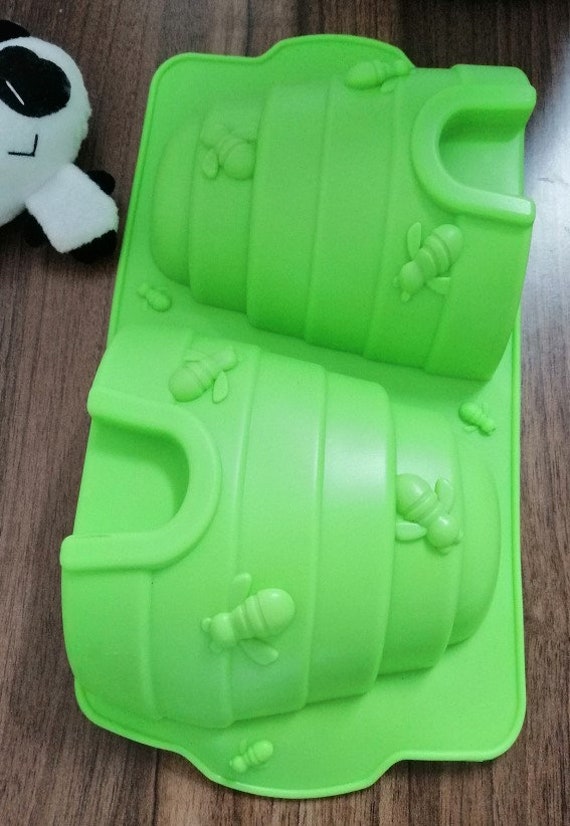In this vibrant, color photograph with a portrait orientation, the subject is a children's sand mold designed to create a beehive-shaped structure. The sand mold is made from lime green plastic and features a two-piece configuration in a single mold. It is rectangular in shape, with handles situated near both the top and bottom for easy use. 

The upper portion of the rectangular mold showcases one side of the beehive, detailed with raised bee figures applied to the exterior, and includes an arched opening towards the bottom. The lower portion mirrors the upper half, offering another identical side of the beehive, complete with the same intricate details.

Partially visible in the top left corner of the image is a white teddy bear, adding a touch of softness to the scene. The entire setup is positioned on a brown wood surface, contrasting with the bright green of the sand mold. The photograph exhibits elements of representationalism realism, capturing every detail with clear, lifelike precision.